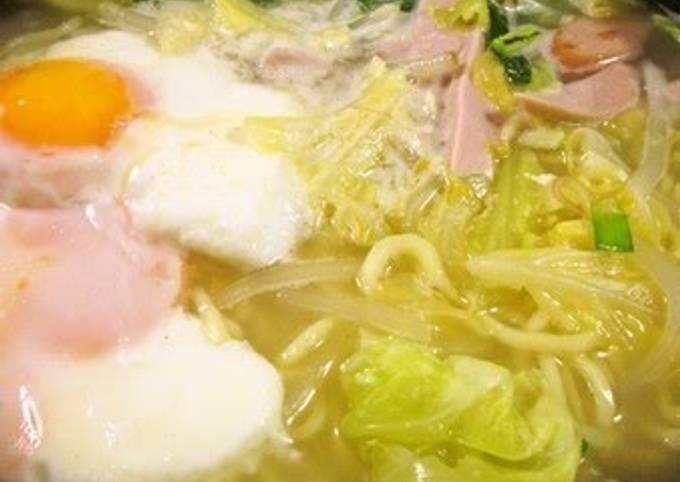The image captures a close-up view of a rich, detailed soup noodle dish. Dominating the dish are long yellow noodles immersed in a pale yellow broth, which appears to be a light chicken broth. In the top left corner, a perfectly cooked sunny side up egg displays its bright yellow yolk melting into the softly solidified white. Below the egg, there is a piece of ham and several pieces of white fish cake. Scattered throughout the dish, you can see tiny green specks of green onion and white onion strips, adding a fresh vibrance to the composition. The top right corner features additional pink slices of ham alongside bright green scallions and leafy greens, possibly cabbage or lettuce, enhancing the visual appeal of the dish. Each component harmonizes to create a visually inviting and scrumptious presentation.